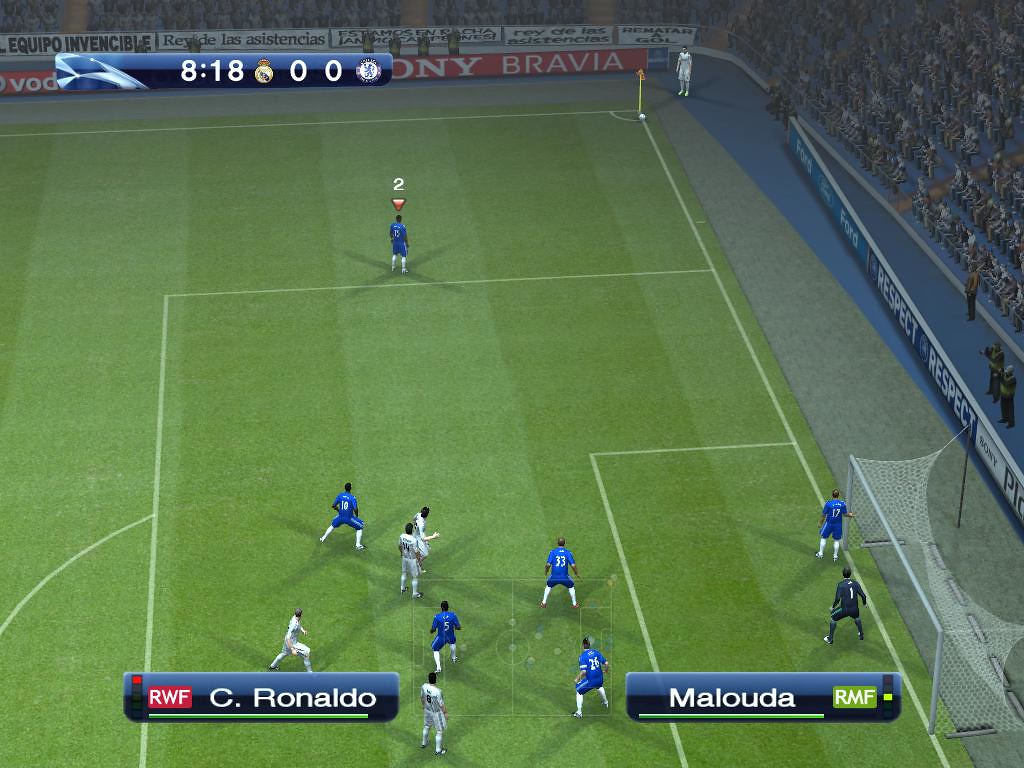In this detailed scene from a FIFA soccer game, the scoreline is tied with Real Madrid and Chelsea both at 0-0. The game time displayed at the top left corner reads 18:18. The selected players, Cristiano Ronaldo and Malota, are shown at the bottom of the screen. The image captures a tense moment as a white jersey player is about to take a corner kick. Positioned in front of the goal, a mix of blue and white jersey players eagerly await the ball. The goalpost is situated in the bottom right, adding to the frame of the picture. To the right, a vibrant crowd of spectators is visible, immersed in the action. The scoreboard and player information reside in the top left and bottom left corners respectively. The lush green field is vividly detailed, with stands full of fans draped in blue on the right side and red on the upper stands. The arena's lights are fully illuminated, enhancing the electrifying atmosphere of the match.